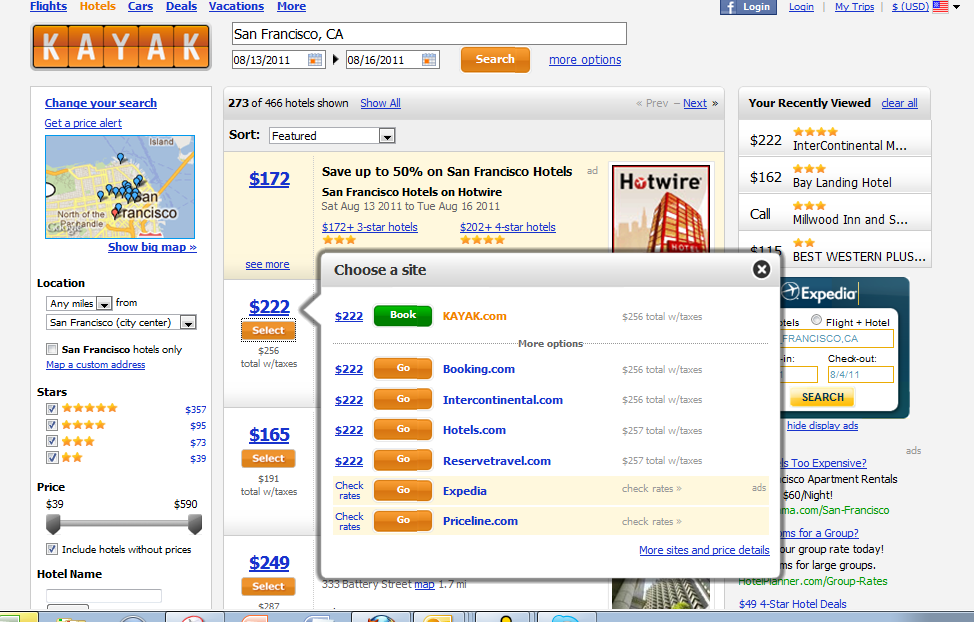This is an image of the front page of a travel company's website. At the top of the page, there is a navigation bar with options for "Flights," "Hotels," "Cars," "Deals," "Vacations," and a "More" drop-down menu on the left-hand side. On the right-hand side of the navigation bar, there are icons and options for Facebook login, "MyTrips," a currency display showing "USD" next to an American flag with a drop-down arrow.

The website's logo, "KAYAK," is prominently featured in the center, with each letter displayed in a separate block with an orange background and white font. Below this, there is a large search bar with "San Francisco, California" entered as the destination. Beneath the location input, there are date fields for selecting travel dates, accompanied by buttons for "Search" and "More options."

Further down, it displays a summary indicating "273 of 466 hotels shown," with the "Show All" option highlighted in blue and underlined. Below this, there are four hotel options listed with pricing details. The first option is priced at $172, the second (highlighted as the selected option) is priced at $222 with an additional button to "Choose a site" and a "Book on Kayak" option. The remaining two hotel options are priced at $165 and $249, each accompanied by a "Select" button.

On the right-hand side of the page, there is a section labeled "Your Most Recently Viewed," displaying details of the user's recent activities on the website.

This well-structured and user-friendly layout allows users to effortlessly search and book their travel needs.